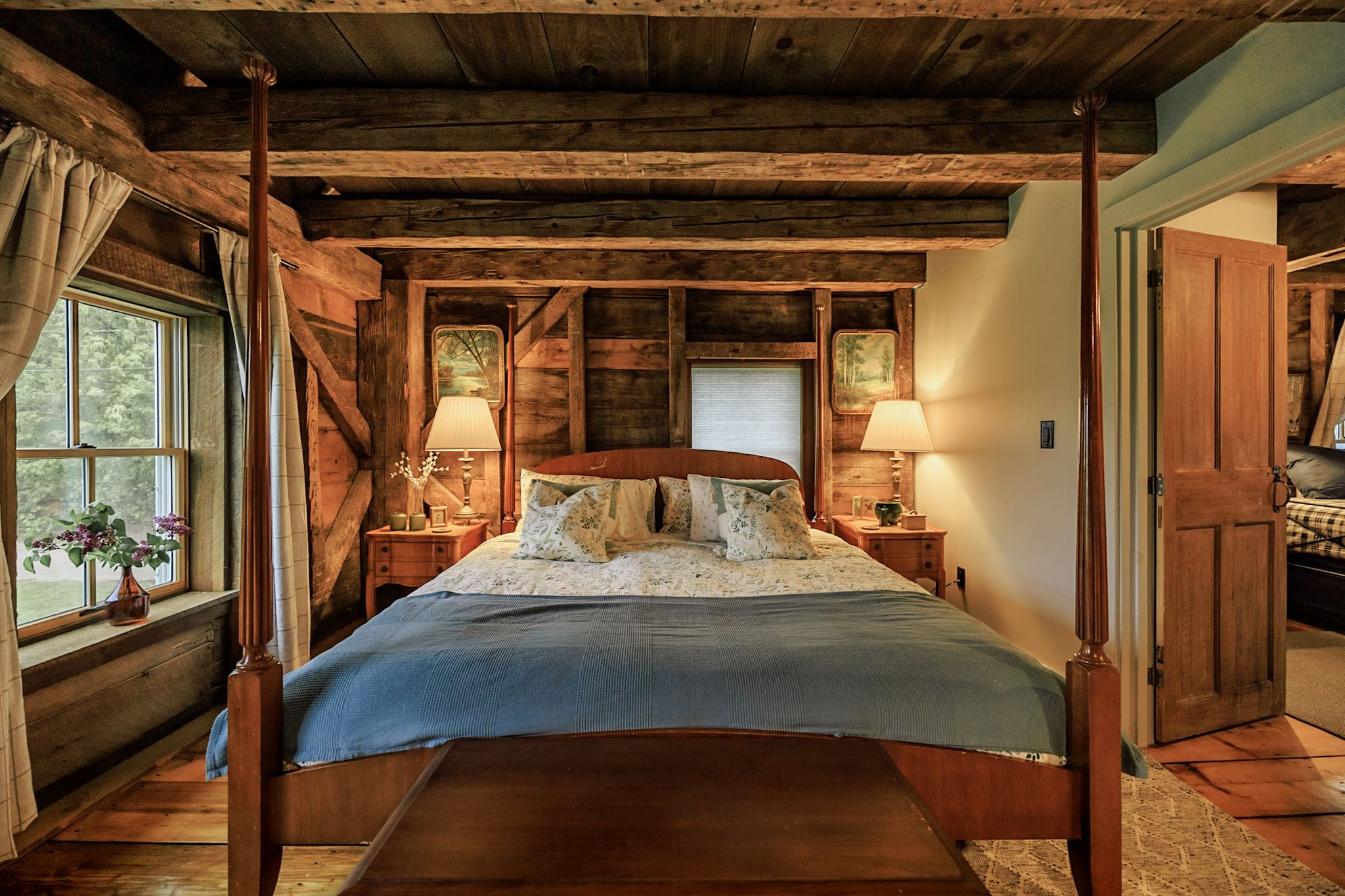This photograph showcases the cozy interior of a rustic log cabin bedroom viewed from the foot of a wooden canopy bed. The bed, dressed with a blue coverlet and a cream and blue patterned bedding, features six plush pillows. On either side of the bed sits a matching wooden nightstand, each adorned with a traditional table lamp and framed art above. 

To the left, a broad window reveals a serene view of trees and a lawn, framed by pushed-back drapery. An amber-colored vase with purple-flowered twigs graces the expansive windowsill. The cabin's structure is characterized by flat timber exterior walls and neatly finished interior walls. On the floor, wide planks are partially visible beneath a cozy rug. 

To the right, an open wooden door offers a glimpse into another part of the cabin. Behind the bed is another recessed window, suggesting a possible extension toward a bathroom. The natural light and warm wooden elements contribute to a welcoming, rustic ambiance.